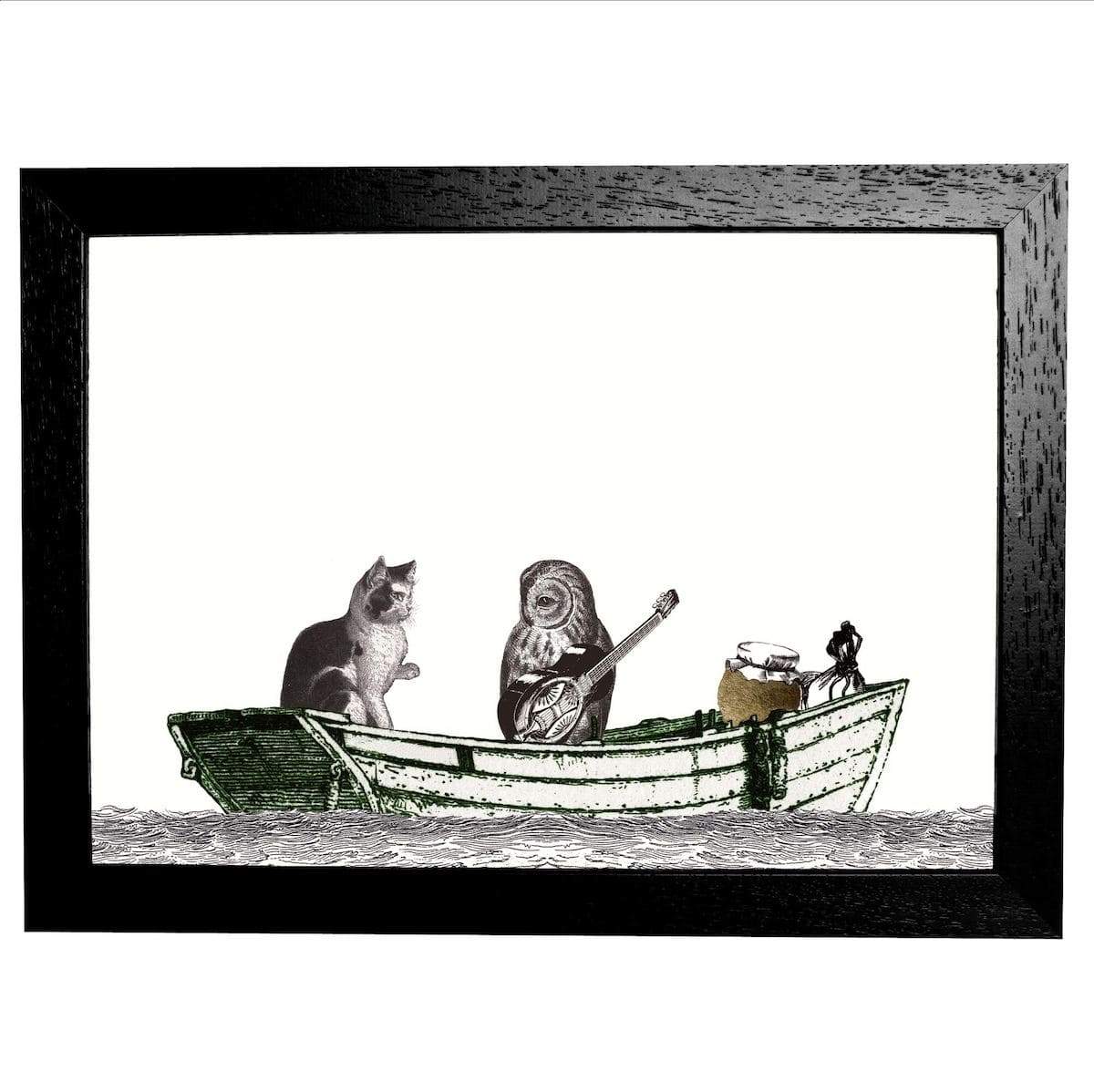The piece of art is an intricately detailed illustration with a mixed-media feel, framed in a black wooden frame, revealing a bit of the wood grain beneath the stain. The background is predominantly white, evoking the texture of canvas or paper, and the scene is in landscape orientation. The focal point lies in a wooden rowboat, featuring bumps, scratches, and dings, and rendered primarily in black and white. Dominating the boat are two central figures: an owl and a cat. The owl, positioned in the middle of the boat, holds a dobro guitar, distinguished by its circular steel resonator, and gazes intently to its right at a black and white cat sitting at the back of the boat with its left paw lifted. The serene exchange between the two creatures is complemented by detailed line work in the water below, depicting gentle waves. Notably, the only splash of color in the illustration is a brown jar covered with a white cloth, tied with a cord, situated to the side of the boat. The overall composition is accentuated by the ample white space in the upper portion of the artwork, creating a harmonious balance.